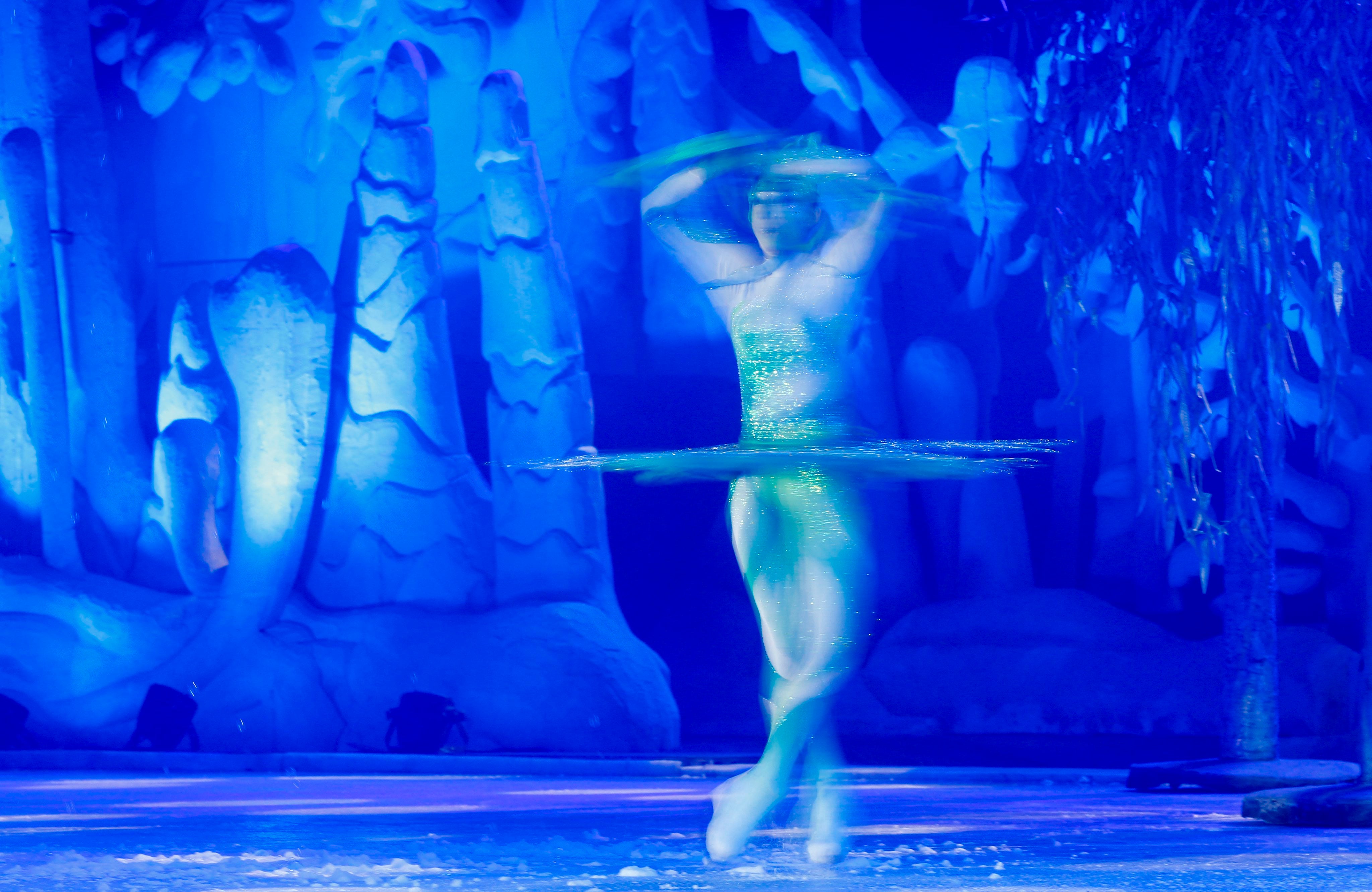In this dynamic, motion-captured photograph, a dancer is vividly depicted in mid-spin, creating a striking image of energy and elegance. She’s gracefully poised on her tiptoes, reminiscent of a ballerina, with her arms held high above her head, appearing slightly blurred due to her rapid twirl. Her voluminous skirt flares out in a perfect circle, adding to the sense of movement, and she’s clad in a green and white outfit with ice skates, suggesting a performance on an ice stage.

The predominant color palette of the image is a deep royal blue, with the ice surface below reflecting bright blue and white highlights. In the background, a serene winter scene unfolds, featuring snow-covered trees and large snow cones, enhancing the chilled atmosphere. The intricate details of ice shavings on the smooth surface beneath her add to the authenticity, further emphasizing the cold, frosty setting of what appears to be an indoor ice rink or stage.